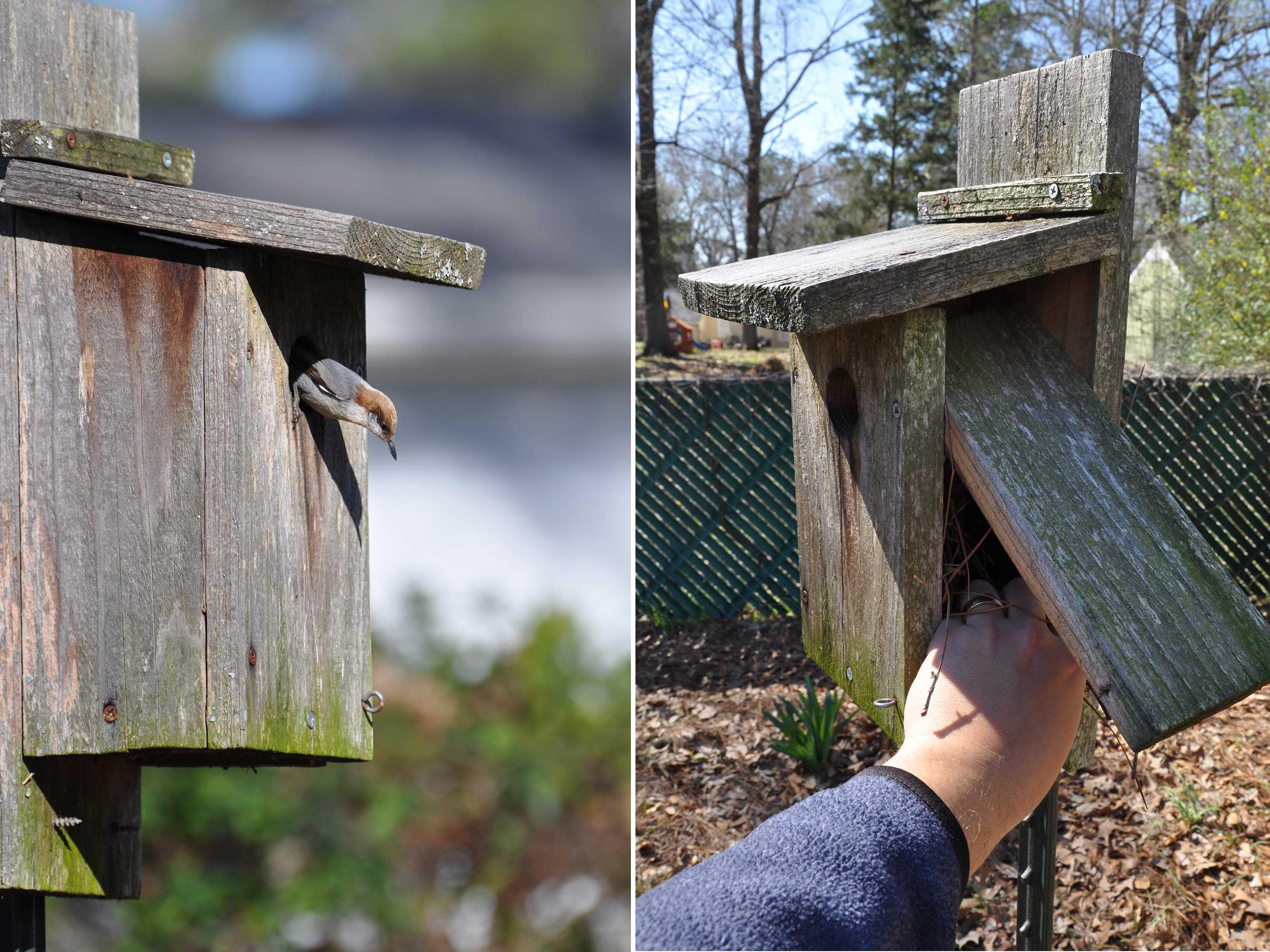The split image showcases two perspectives of an aged wooden birdhouse. In the left photograph, an older birdhouse perched on a post is detailed with green moss and rusted nails. A small bird, featuring a predominantly gray body, white under its chin, a dark beak, and a brown spot on its head, pokes its head out of the entrance hole, gazing downwards. The blurred background transitions from greenery at the bottom to gray hues at the top.

In contrast, the right photograph captures a side view of the same birdhouse, revealing its inhabited nest through an open side plank. A hand clad in a blue fleece reaches inside, presumably to inspect or fix the nest. Surrounding the scene are dry leaves on the ground, a small fence, a chain-link fence with green privacy slats, and various trees in the distance, some bare and others partially leafed, alongside a tall pine tree. The background is further highlighted by a clear blue sky.